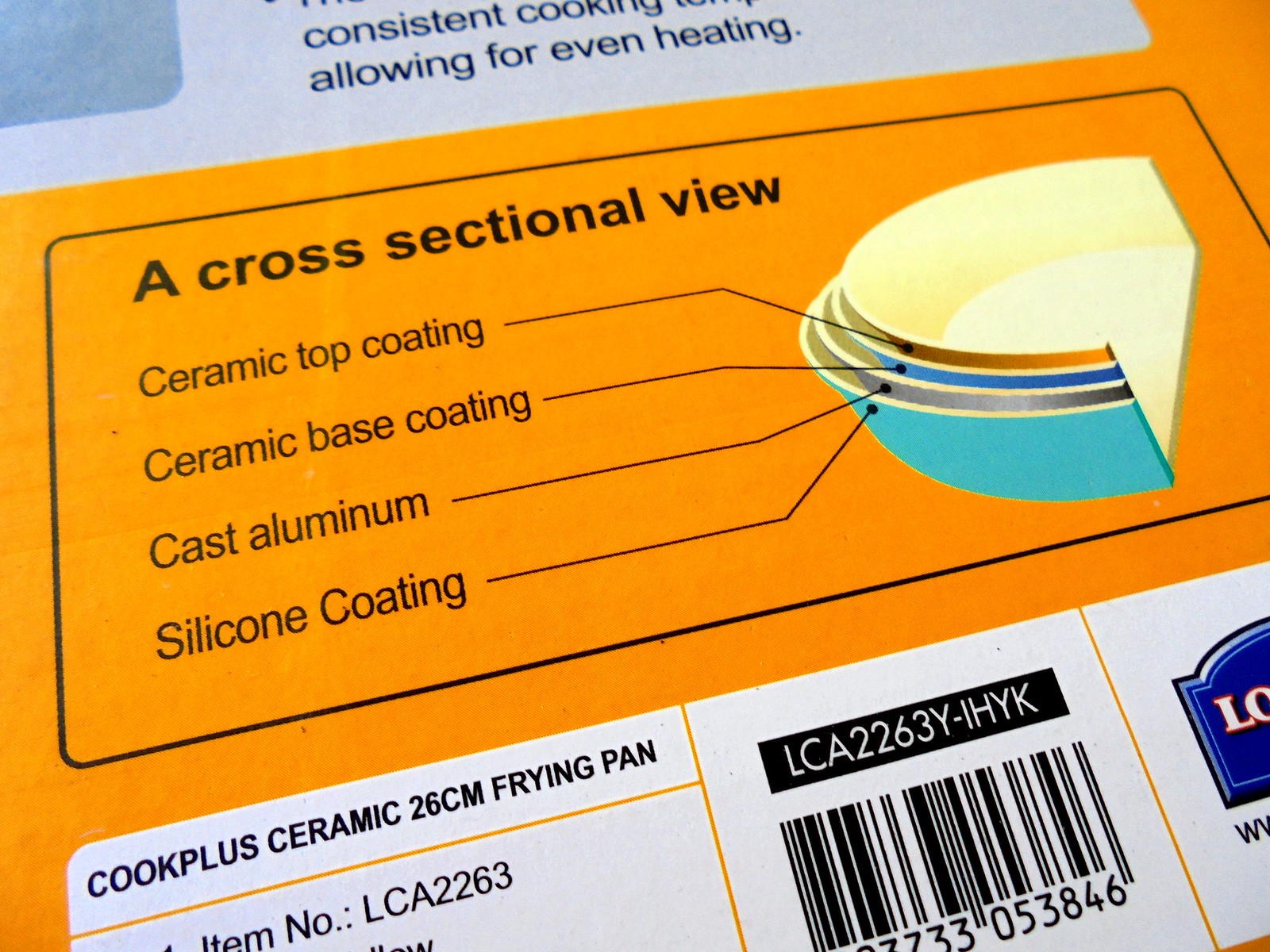This image appears to be a close-up of a product label on a frying pan box. At the top left, there's a blue, rounded rectangle with partial text indicating "consistent cooking, allow for even eating" written in black on a white background. Below this, the prominent orange section is bounded by thin black lines, framing a black rectangle with rounded corners. The text "A cross-sectional view" is prominently displayed within this black rectangle. Below this header, an illustration depicts a half-oval shape representing the frying pan's layers, with yellow-edged slices. Each slice is color-coded in teal, green, gray, blue, and goldish brown. Labels with arrows pointing to these slices denote "ceramic top coating", "ceramic base coating", "cast aluminum coating", and "silicone coating". Further down, more labeling on a white background includes "Cook Plus Ceramic 26CM Frying Pan, Item Number LCA2263". Adjacent to this, there's a barcode with numbers underneath, partially occluded text, and a small blue symbol featuring reddish outlines of the letters "OL" and possibly "WV".